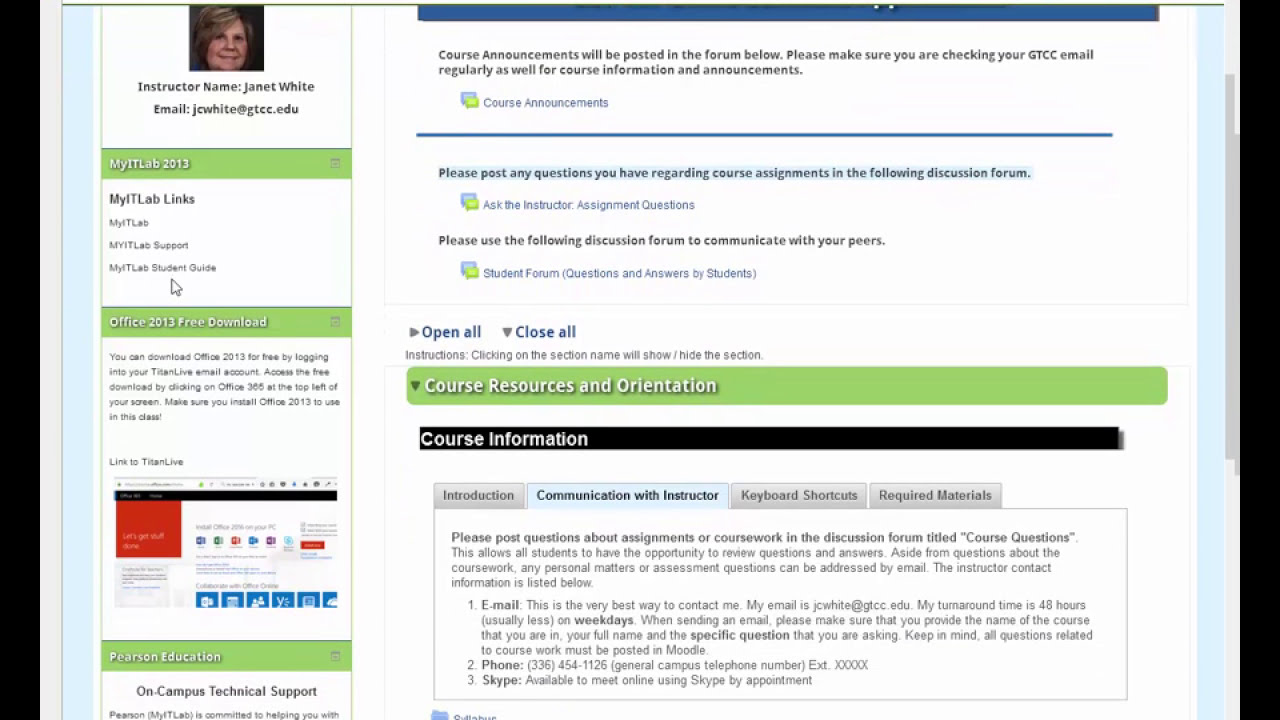This image is a detailed screenshot of a web page for an online course, presumably part of a school website. At the upper left corner, there's a small photo of the instructor, Janet White, who appears to be a woman in her 50s or 60s with blondish hair with streaks. Her name and email (jcwhite@gtcc.edu) are positioned next to the image. The page features multiple sections and colorful boxes containing various course-related information. Notably, there are sections labeled "My IT Labs Link," "Office 2013 Free Download," "Pearson Education," "On-Campus Technical Support," "Course Announcements," and "Course Information." The layout uses a palette of colors including red, blue, green, white, black, gray, and a bit of purple. A large blue rectangular shape spans the top of the page. Text and announcements are positioned throughout, encouraging students to check their gtcc email regularly for updates. Additional links and resources are organized within the sidebar and main content area, guiding students through the course material and available support services.